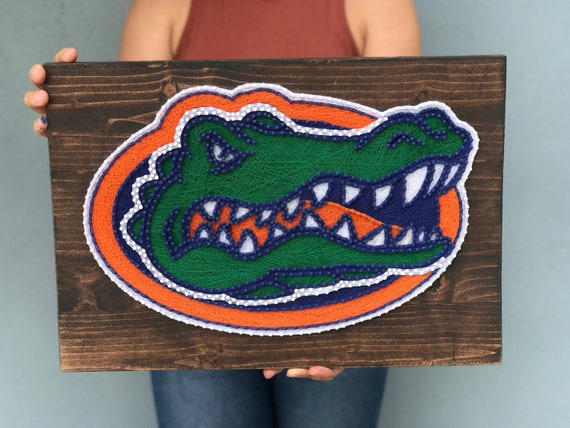In front of a light blue background, a woman is pictured holding a dark brown wooden sign. She is dressed in a little red tank top paired with blue jeans. The sign she holds, with one hand at the top and the other at the bottom, prominently features the Florida Gators logo. This logo showcases a large green alligator with a fierce expression, displaying sharp white and orange teeth and a menacing eye. The alligator is set against an orange and blue background, which are the official colors of the University of Florida. The gator's open mouth and aggressive demeanor suggest it is ready to take a bite out of something, embodying the spirited competitiveness of the Florida Gators.